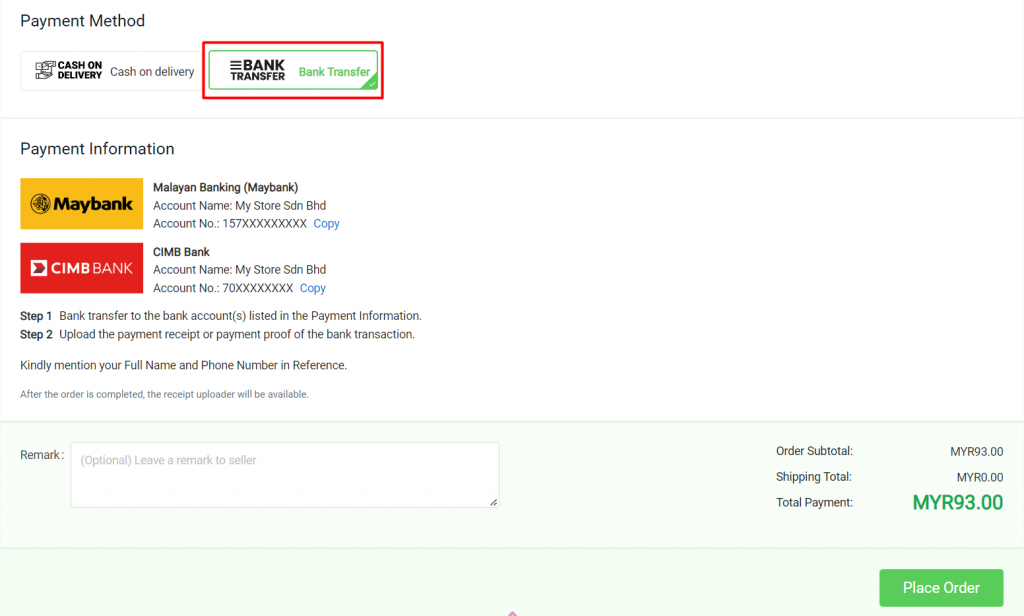This image is a screenshot of a payment summary for a bank transfer. In the top left corner, two buttons are visible, immediately indicating the presence of payment options. The section header "Payment Method" clearly signifies that this document pertains to a payment summary. Below the title, there are two notable buttons: the first on the left depicts "Cash on Delivery" with an icon symbolizing a cash exchange, while the button on the right is highlighted with a green border indicating "Bank Transfer," which is the chosen option. Additionally, a red border around the "Bank Transfer" button suggests this guidance is part of a tutorial instructing the user to select this method.

Proceeding downwards, the "Payment Information" section presents details with two bank logos. The first logo, in yellow, belongs to Maybank, specified as Malayan Banking (Maybank). It lists the account name "My Store SDN BHD" with an associated account number and includes an option to copy these details. The second logo, in red, represents SimBank, which also offers the same account name but with a different account number.

Following these details are two steps instructing how to transfer the payment to the appropriate bank account, accompanied by an option to upload a transaction receipt or proof of payment. Towards the bottom left, there is a blank field labeled "Remark to Seller" where users can leave comments or special instructions.

On the bottom right, there's a section displaying the payment summary, which includes the order subtotal, shipping cost, and the total payment amount displayed in green, which is MYR 93.00. Finally, a prominent green "Place Order" button is located at the bottom right to finalize the transaction.